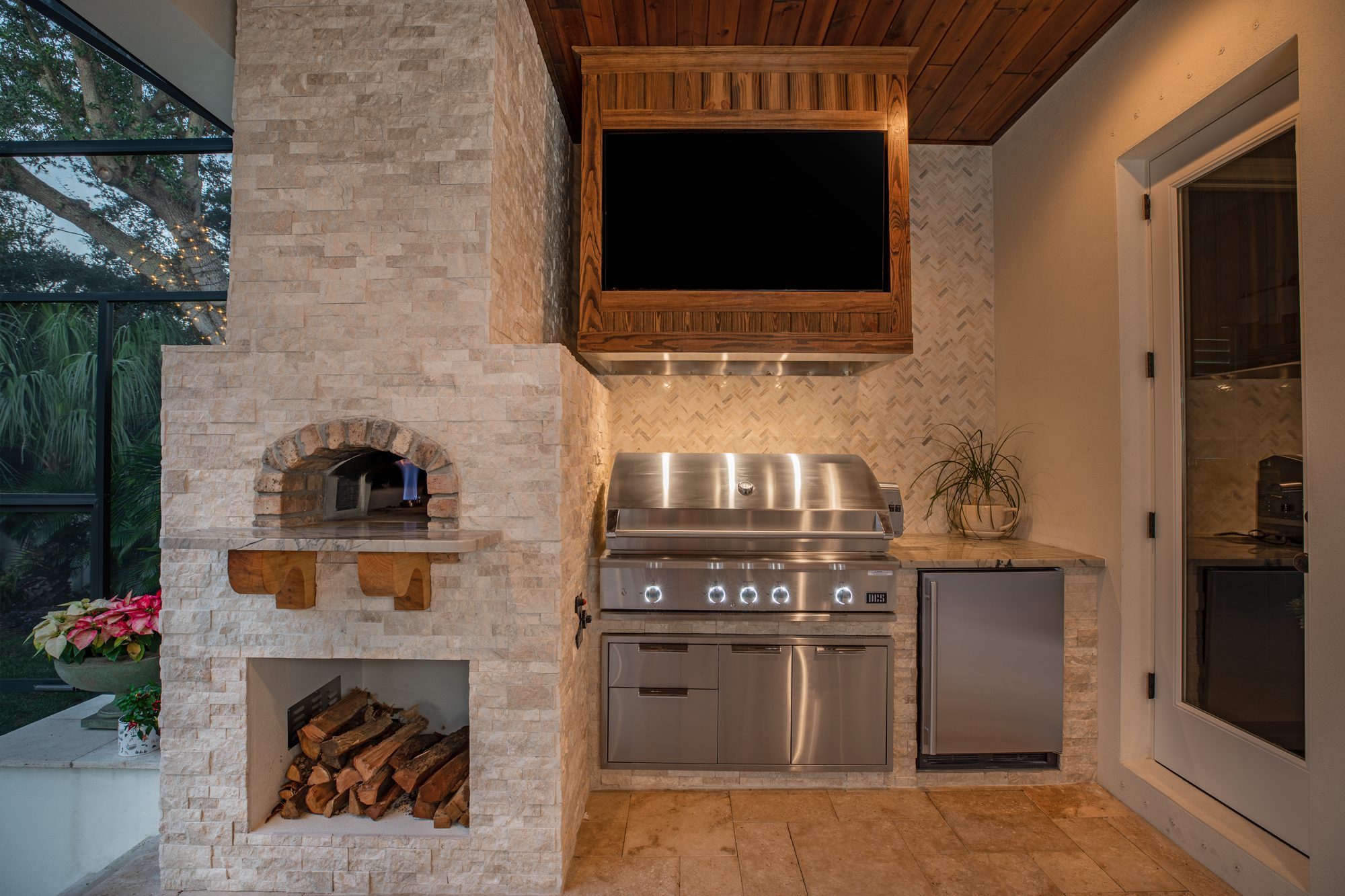This photograph captures an enclosed patio-like kitchen space, possibly part of a sunroom. On the left, a large glass section with black rectangular frames offers a view of outside trees and foliage. Pink, yellow, and white flowers are placed inside this glass section, adding a touch of nature indoors. To the right of this is a substantial brick structure, made of light-colored, beige bricks, housing a traditional wood-fired pizza oven. Neatly stacked logs for the oven are stored underneath the brick pillar, which has an opening for inserting pizzas.

In the central area of the kitchen, there is a large stainless steel stovetop or range, featuring five control knobs and various buttons. Above the range is what appears to be a TV screen, encased in a wooden frame, providing a modern touch to the rustic setting. The floor in front of the cooking area is made up of brown stone-like tiles, and natural light illuminates the space.

To the further right, there's a small stainless steel appliance, either a mini fridge or a dishwasher. Adjacent to this appliance is a large glass door framed with wood, which presumably leads into the main part of the house. The overall design of this space is ornate and thoughtfully integrated with both contemporary and traditional elements.